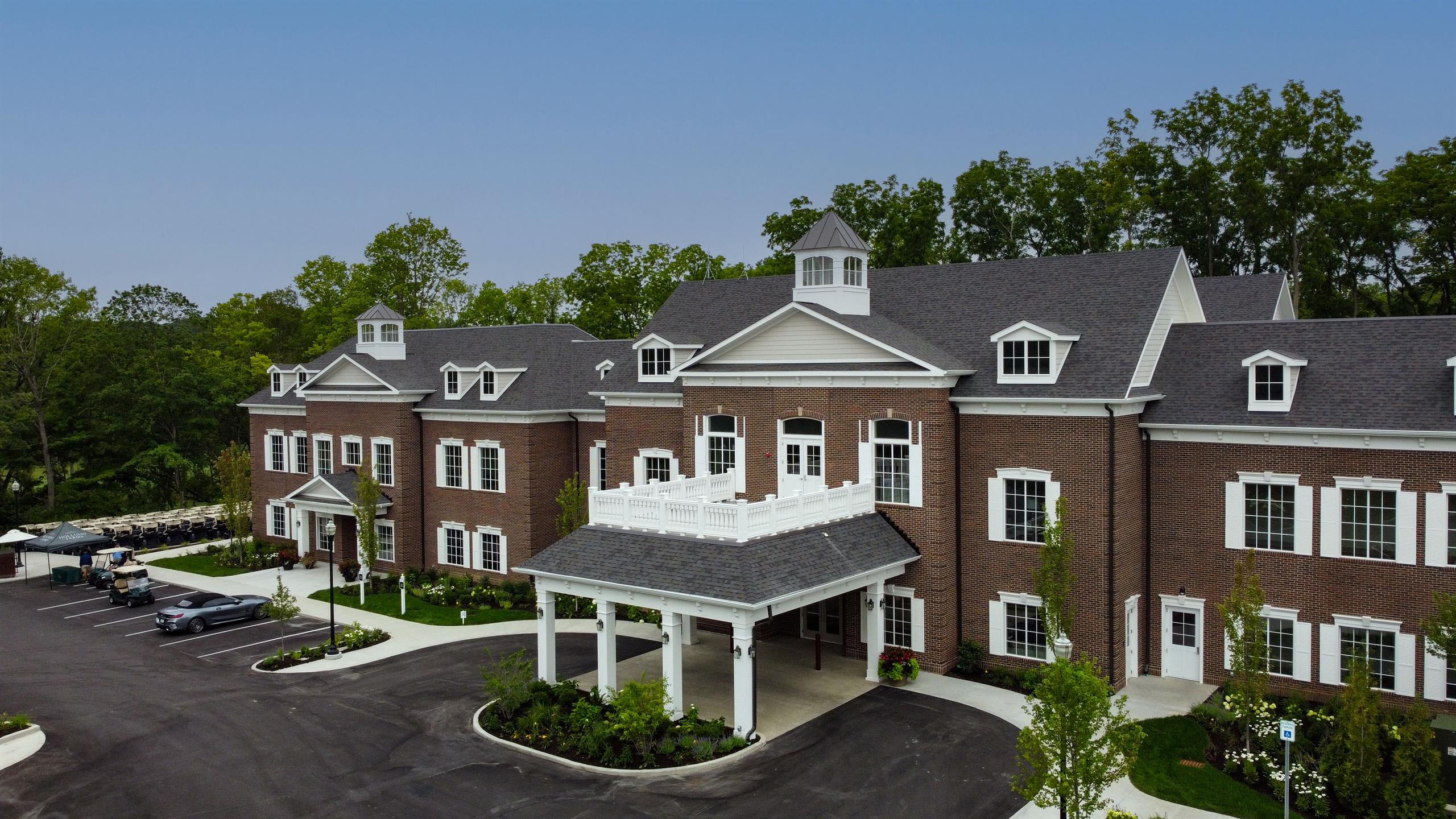The image depicts a sprawling country club or estate building made of dark brown brick with blue shingles on its roofs and an array of white windows, each adorned with white window slats on either side. This grand structure is composed of three connected buildings, each standing three stories tall. At the center of the main building, there's a large entrance with a prominent silver-topped roof, supported by white columns, providing an overhang for vehicles. Above this entrance, there's a balcony enclosed by a white fence. In front of the entrance is an enclosed area lush with green plants and young trees. On the left side of the image, a small parking lot hosts a luxury convertible car, two golf carts, and several other vehicles. The scene is set on a clear, sunny day under a vibrant blue sky, with additional details such as well-kept grass, trees, and various minor structures including tents and arranged chairs visible in the background.